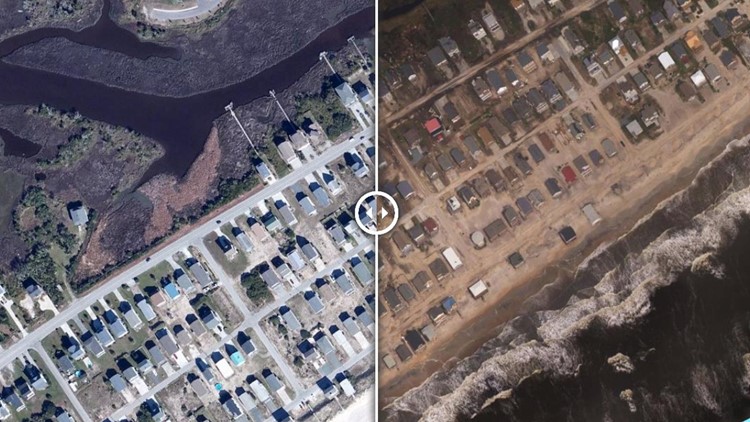This detailed satellite image is divided into two parts by a vertical white line with a circular control in the middle, featuring arrows for sliding between the two views. The left side of the image showcases a developed suburban area with regularly spaced houses featuring blue and white roofs, interspersed with paved roads in gray and fields in dark brown. The diagonal orientation of the road starts from the bottom left and stretches to the middle and bottom right of this section. Above the road, there are additional land areas and possibly a water body.

On the right side, the image depicts a coastal region with sandy soil displaying a classic yellowish-brown color. This area contains numerous houses with roofs in a variety of colors, ranging from white and red to brown. The beach is clearly visible with the ocean waves lapping at the shore on the bottom right side, and a diagonal stretch of both sandy and residential areas extending from the bottom left to the middle right. This comparative visual suggests a transformation over time from a beach area to a developed suburban environment.